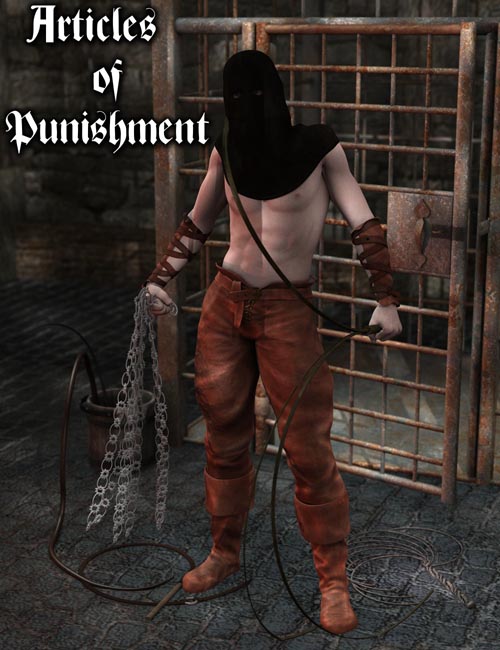The image resembles a screenshot from a video game, set in a dungeon with a dark, foreboding atmosphere. The scene features a shirtless man standing on a gray cobblestone floor, with a large, rusted jail cell in the background; its door is slightly ajar. The man wears a black hood covering his head and shoulders, leaving only eye slits visible. His arms are stretched out to his sides, and both forearms are wrapped in dark brown leather straps. He holds a whip in his left hand, draped over his shoulder, and in his right hand, he grasps a weapon adorned with five hanging chains. Completing his menacing appearance, he wears brown pants and boots. Nearby, there is a bucket filled with additional whips, reinforcing the dungeon's oppressive vibe. In the upper left corner, text in white letters with a black border reads "Articles of Punishment," indicating that this area is designated for meting out punishment.